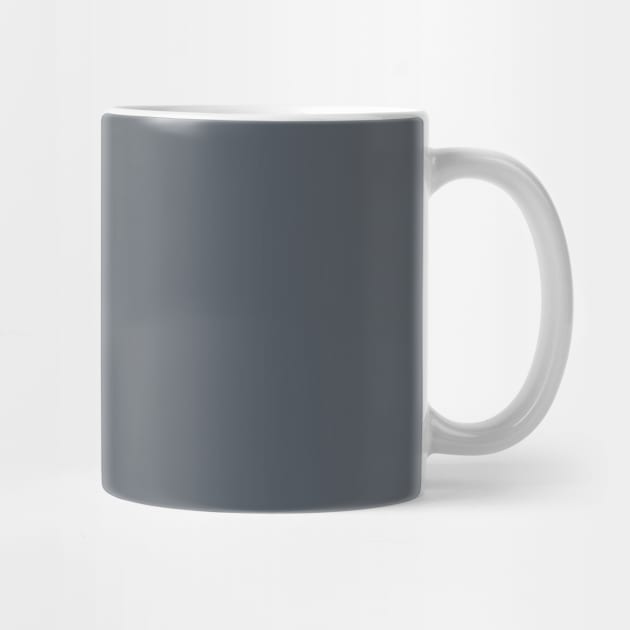The image depicts a modern, standard-sized coffee mug set against an all-white background. The mug features a dark gray, cylindrical exterior with a glossy finish and a white rim, which reflects the light subtly. Its handle is a slender, reverse C-shape, also in white, seamlessly attached to one side. The interior of the mug mirrors the white color of the handle and rim. This everyday pottery mug stands approximately four to five inches tall, exhibiting a sleek and plain design, devoid of any imperfections or artisanal touches, indicative of factory production. The bright white background further accentuates the simplicity and elegance of the mug's two-tone color scheme.